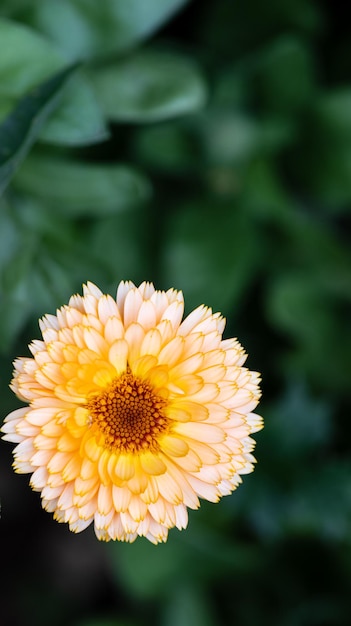This color photo, captured in portrait mode, showcases a close-up of a vibrant chrysanthemum flower set against a dark green leafy background. The flower's numerous petals transition from a soft, pale pink at the edges to a light yellow towards the center. These petals are arranged in overlapping layers, creating a textured and visually captivating bloom. The core of the flower is a vivid brownish-orange, dotted with tiny pollen bearers. The background consists of out-of-focus leaves and stems, with dark green palm fronds providing a contrasting backdrop that emphasizes the sharp detail of the chrysanthemum's burst of colors.